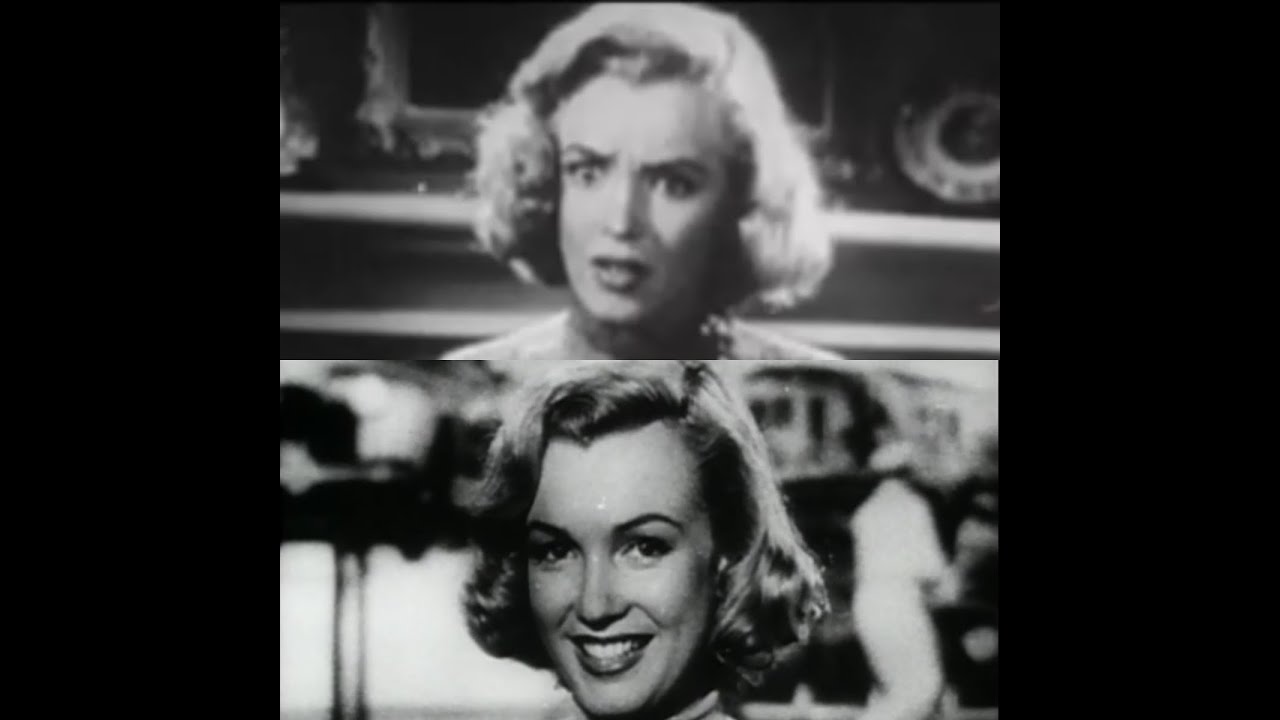The image depicts two side-by-side, black-and-white photographs of a young, light-skinned woman, arranged with one on top of the other. The top photograph is noticeably blurry, possibly an original, lower-quality scan from an old movie or commercial, and shows the woman with white hair looking slightly scared and confused, directly at the camera. The clarity is poor, making her features less distinct. Below, the bottom photograph appears to be a higher-definition rendition, much brighter with improved white opaqueness and greater detail. In this image, the woman is smiling, revealing her teeth which shine through the grey scale of the black-and-white format, and she is wearing lipstick. The bottom image shows the woman slightly older and more content, with more distinct features including her nose and mouth. Both images are framed by black vertical bars on either side, creating a uniform format. There are indistinct, blurred backgrounds in both photographs, emphasizing the woman as the primary focal point. The comparison suggests an attempt to illustrate the difference in image quality, potentially highlighting a restoration or upscale to a modern, higher resolution.